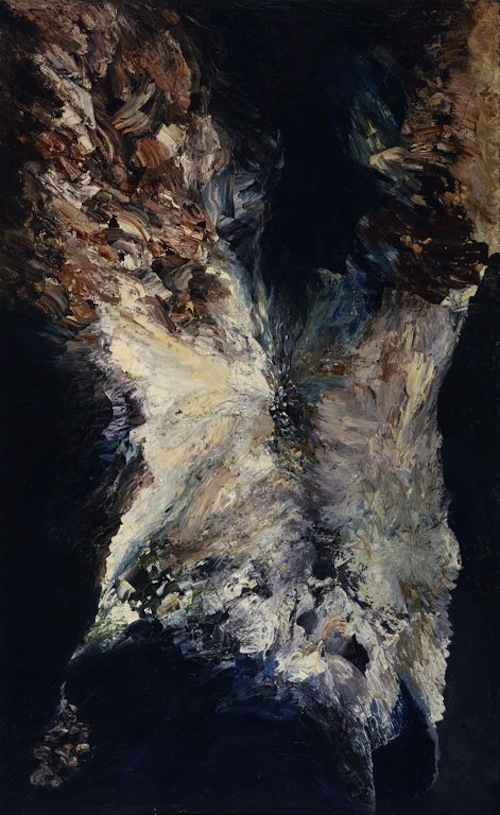This abstract painting, titled *The Annunciation*, is a striking vertical rectangle dominated by a dark, almost black background speckled with faint gray and white dots. The artwork displays a dramatic interplay of contrasting colors and textures, creating a rock-like surface that transitions from deep, uneven dark blue with gray areas at the bottom to a lighter, more varied palette as it ascends. The central section features dynamic brush strokes in white, gray, green, and light brown hues, evoking a sense of motion and depth.

As the painting progresses upwards, it morphs into jagged areas with wooden tones interspersed with creamy smears of paint. This mix of colors branches out into a V shape or heart shape, with the brown smears blending with the creamy whites. On the left side, the wooden colors cut into the black background, creating a jagged and uneven appearance, echoing the feeling of carvings. Adjacent to this is a pitch-black segment with bluish tones, intensifying the depth perception. 

The dabbled, dashed brush strokes give an impression of motion, like looking down at a river, and suggest a faint resemblance to a female figure. The painting's intricate details and abstract nature invite various interpretations, blending extreme detail with a profound sense of abstraction.